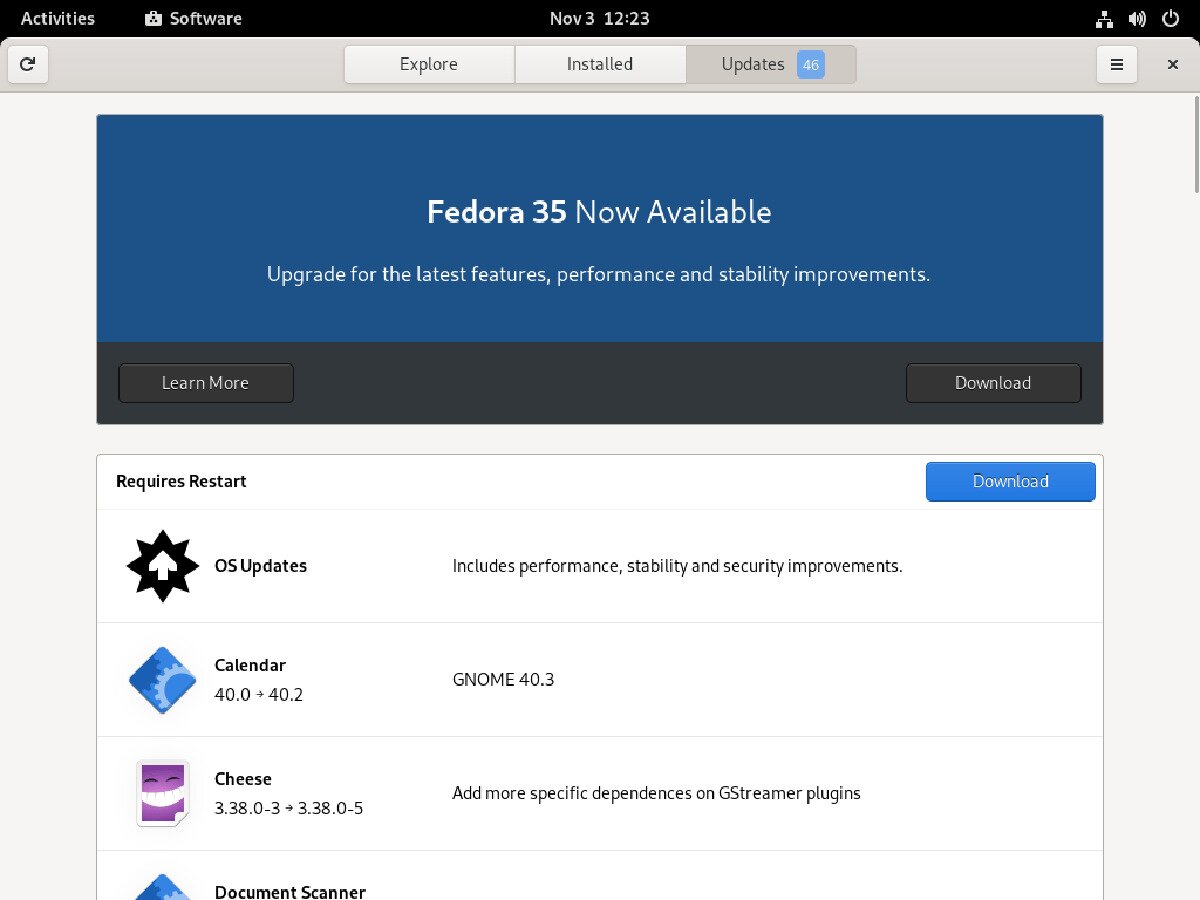**Detailed Caption:**

This landscape-oriented screenshot captures an update notification for Fedora 35. At the top left corner, the interface displays a black strip with the option "Activities" and the label "Software" partially visible. The header in the upper center reads, "November 3rd, 12:23." Below this is another black strip with a blue background and a prominent message indicating, "Fedora 35 now available. Upgrade for the latest features, performance, and stability improvement."

Proceeding downwards, a black stripe on the left side has the option "Learn More," while on the right, it has a "Download" button. Directly beneath, against a white background, there is an advisory stating, "requires restart" on the left, accompanied by a blue "Download" button on the right.

Following this, a section outlines the OS updates which include enhancements for performance, stability, and security. The next row lists specific software updates, starting with "Calendar 40.0 to 40.2," followed by "GNOME 40.3," and "Cheese 3.38.0." Additionally, there are notes about specific dependencies additions for GStreamer's plug-ins.

Overall, the screenshot emphasizes the available upgrade to Fedora 35, essentially offering users options to explore the new features, install updates, or begin the upgrade process.